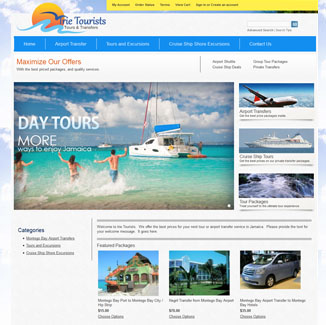Screenshot from a travel website titled "The Tourists Tours and Timeshare." The main feature of the website is a somewhat blurry photograph of a boat with its sail down, anchored near the shore. Three individuals are seen running through the ocean toward the boat. The caption at the top reads: "Day Tours - More Ways to Enjoy Jamaica." On the right-hand side of the website, there are additional images including an airplane in flight, a cruise ship, and a body of water, though some details are unclear due to blurriness. Below the main photograph, there is a section titled "Categories," but the specific text is unreadable. Further down, there is a photograph of a building by the ocean, presumably a hotel, alongside an image of a vehicle.